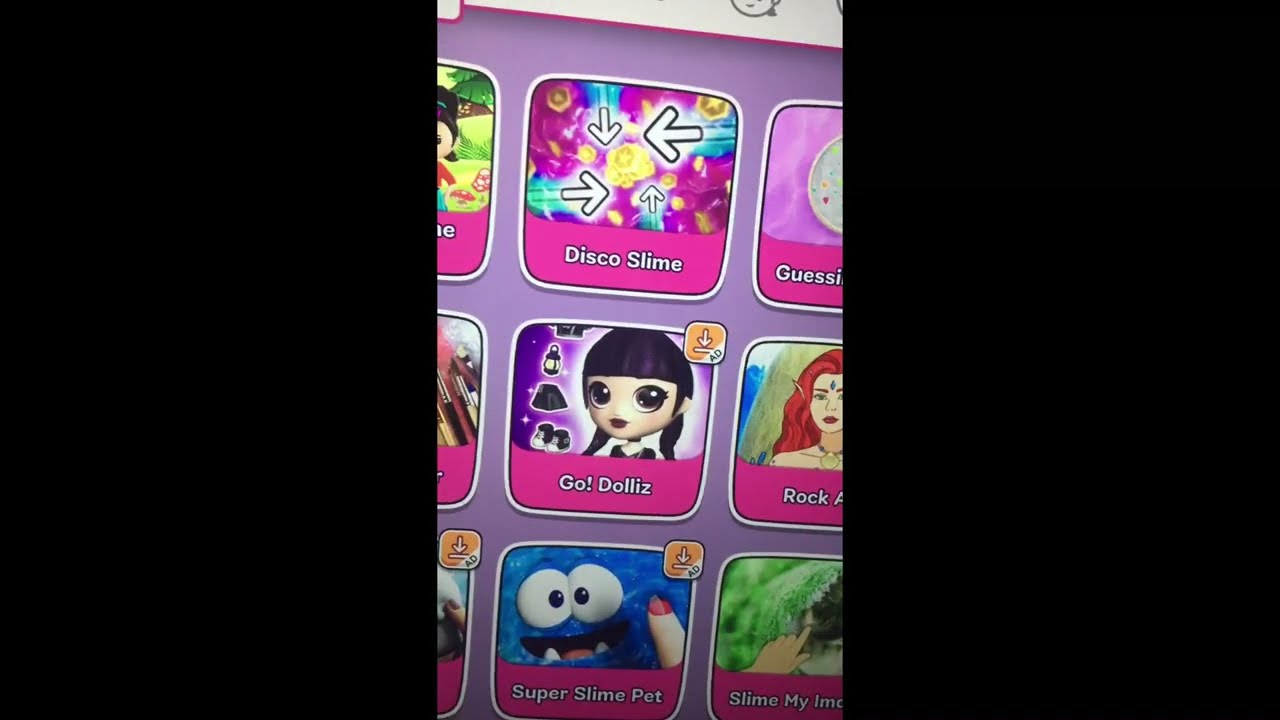The image is a screenshot of a mobile device’s screen displaying a 3x3 grid of app icons, primarily geared towards children's games. The central portion is fully visible, while the apps at the edges are partially cut off. Each icon is contained within a small square, and the screen's background is purple. 

At the top center, there is an app titled "Disco Slime" with multiple arrows around it. To its immediate right, another app icon reads "Guess, Guess, Guess," but is partially cut off. Below "Disco Slime," a pink-background app labeled "Go Dollies" displays a cartoon character with clothing accessories and an "Add" symbol in its top right corner. Adjacent to it is an app titled "Fantasy Woman," featuring a red-haired elf character.

In the bottom row, directly beneath "Go Dollies," is the "Super Slime Pet" app showing a card-animated face and a finger. Next to it is "Slime My LMO," which appears green with a hand icon. Other visible titles include "Rock," "Slime," and potentially "My."

The image's layout and the type of icons suggest it might be from a child's tablet or smartphone, indicated by the playful themes and designs of the apps. At the top and right edges, there are elements resembling typical smartphone iconography, like a download symbol and arrows, suggesting this could be a screen capture from a content-sharing platform like TikTok.